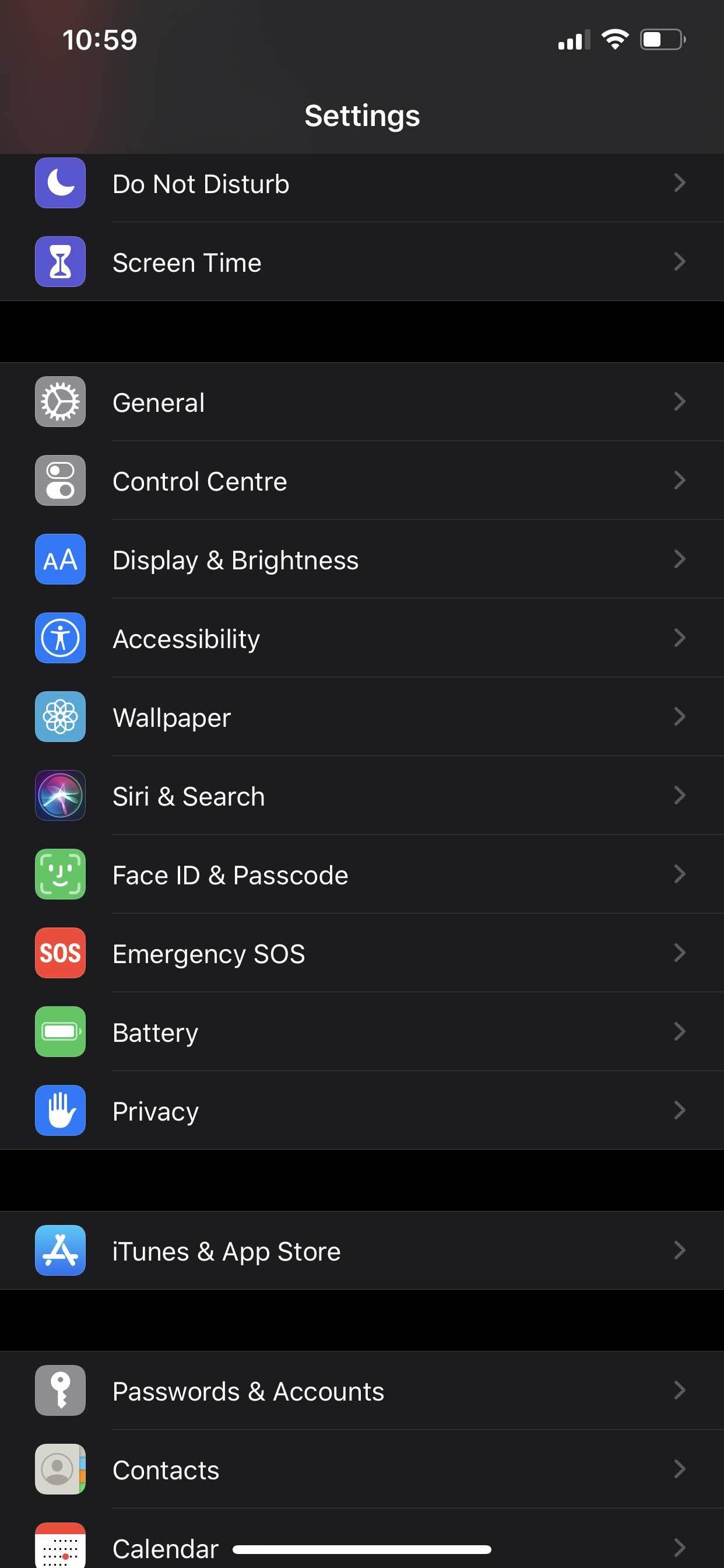The image depicts a screenshot of the settings menu on an Apple device. At the very top, the heading "Settings" is prominently displayed. Below this, a list of options is shown, arranged vertically in sections. The visible options, listed in order from top to bottom, are: "Do Not Disturb," "Screen Time," "General," "Control Center," "Display & Brightness," "Accessibility," "Wallpaper," "Siri & Search," "Face ID & Passcode," "Emergency SOS," "Battery," "Privacy," "iTunes & App Store." Another section below lists more options, including "Passwords & Accounts," "Contacts," and "Calendar." Some of the lower words are partially obscured and cannot be fully read. The time displayed at the top of the screen is 10:59 AM, and there are icons visible on the left side of the top bar, including signal strength, Wi-Fi connectivity, and battery status.